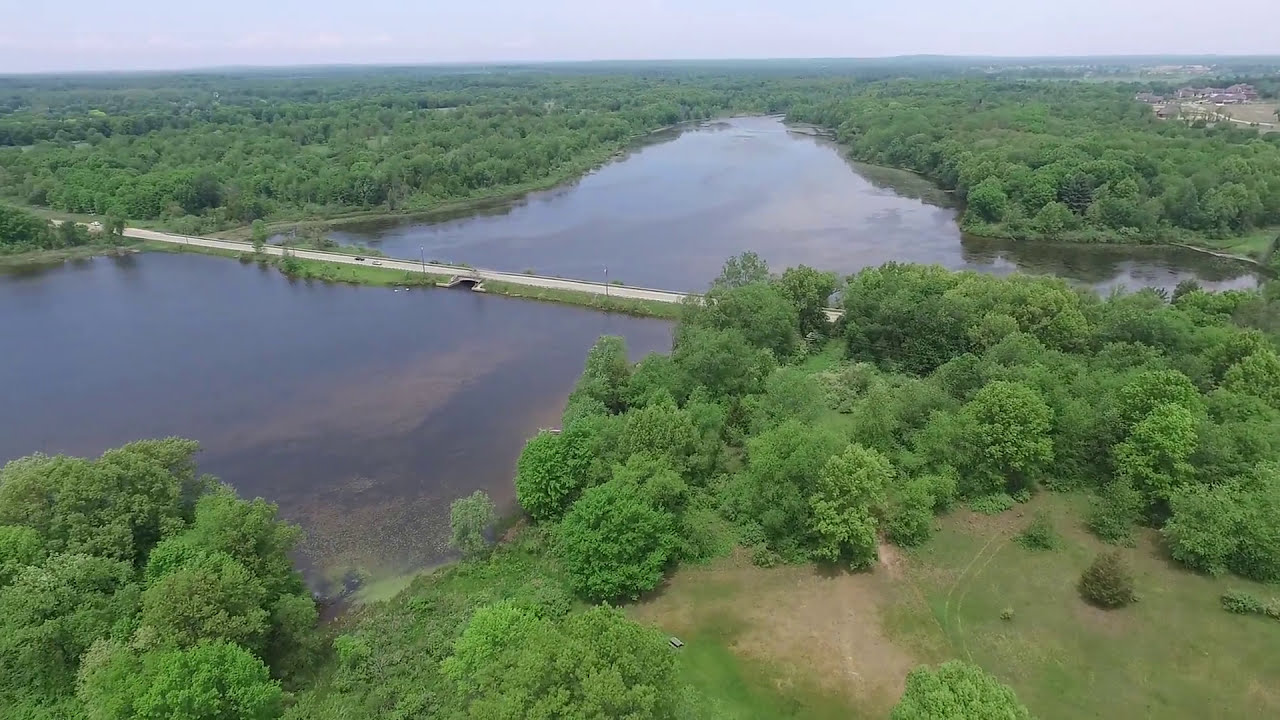This detailed aerial photograph captures a serene landscape featuring a clear river or lake surrounded by plush greenery. Both sides of the water are heavily wooded with vibrant, lush green trees and grassy areas. A two-lane paved bridge, noticeable by the vehicles on it, spans across the water, creating a peninsula-like formation with its road and bridges. The water is clear in some areas, revealing rock shelves and the bottom of the river. In the distance, behind the dense foliage, lies a small neighborhood comprising houses and possibly a barn. The terrain is flat, and the image is capped by a hazy, light blue sky with a few clouds, highlighting the natural tranquility and the subtle human activities blending into the landscape.